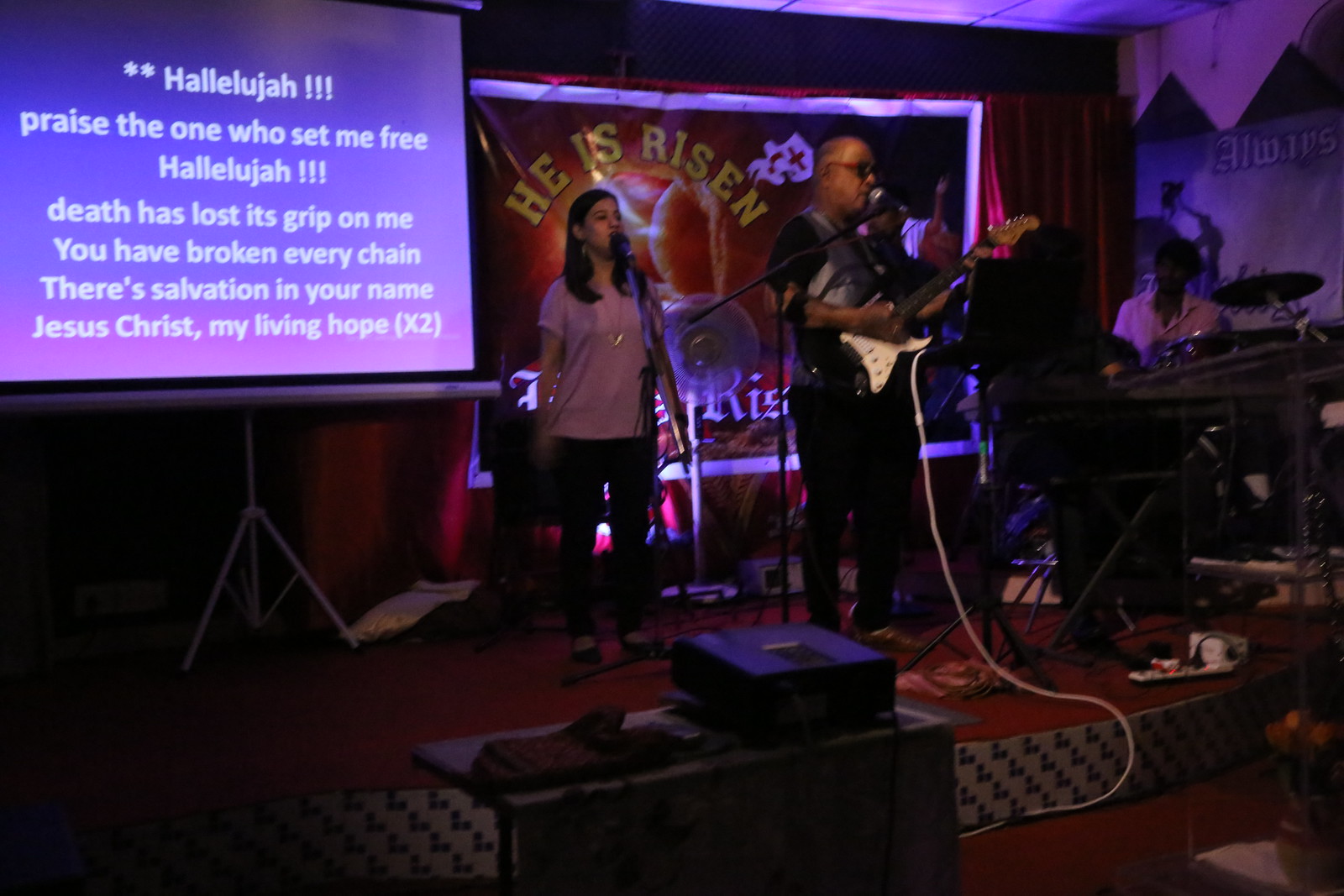In this detailed indoor image taken at a religious concert, we see a central stage with a carpeted floor. At the heart of the scene are two main performers: a man with an electric guitar, wearing sunglasses, positioned directly in the center, and a woman in a white t-shirt and black pants, standing slightly behind him, singing into a microphone. The guitarist is plugged into an amplifier, and a drum set with a drummer is visible to their right. Behind the performers, a red and white banner with yellow lettering prominently reads "He is Risen." To the left, a white projection screen on a purple background displays the text: "Hallelujah! Praise the one who set me free. Hallelujah! Death has lost its grip on me. You have broken every chain. There's salvation in your name. Jesus Christ, my living hope" (X2). The stage is adorned with various colored lights and speakers, contributing to an atmosphere filled with purple, pink, white, gray, red, yellow, and tan hues.